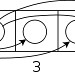This is a highly detailed description of a very small, square photographic image predominantly in white and black hues. The image contains a grid-like pattern composed of square boxes, each outlined in black. Within these squares, there are small circles that appear partially cut off at the sides due to the limited dimensions of the photograph. At the bottom of the central square, the number "3" is clearly indicated. Additionally, two arrows are drawn, pointing upwards directly towards the middle of these circles. An unclear line descends over the middle square, its path uncertain as it may loop back, but this detail is indistinct due to the image's small size. Consequently, many finer details are obscured. The overall composition of the image is simple and minimalistic.